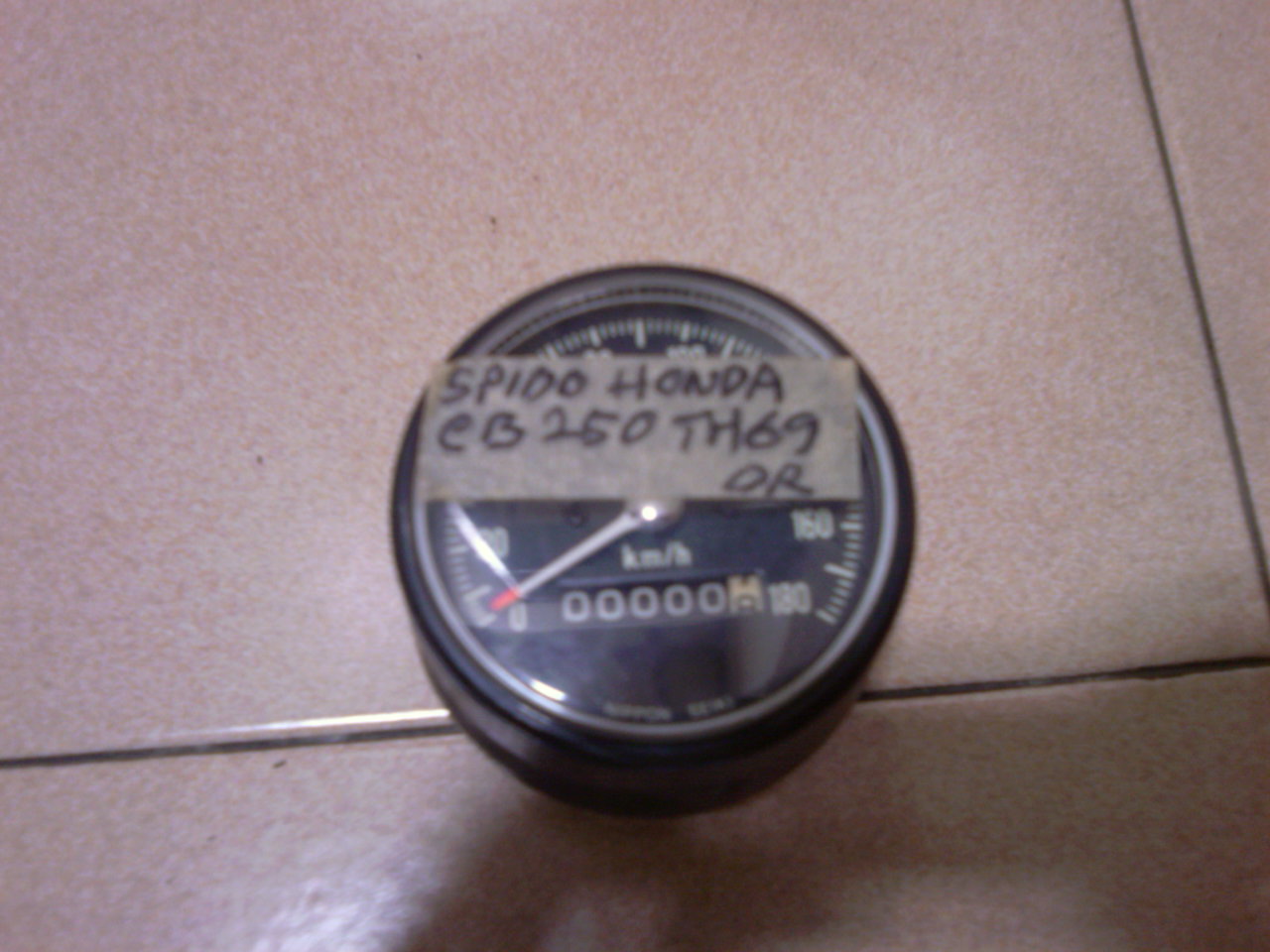This photo captures a detailed view of a thermostat with several unique features. The thermostat, primarily black and cylindrical, prominently displays buttons labeled "PIO," "HANTA," and "EB." It is mounted onto a thermometer gauge, although visibility is somewhat obscured by a piece of masking tape adhered to the device. The entire assembly is situated against the mortar in a strip of tiles, suggesting a tiled surface in the background. Additionally, the thermostat features tick marks, adding to the instrument's functionality and complexity. The photo provides an intriguing glimpse of this precision tool in an applied setting.